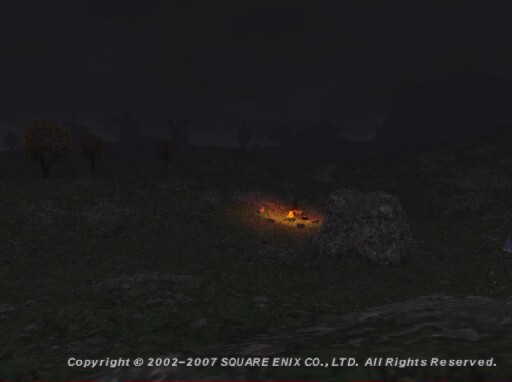A screen capture from an early 2000s to 2010-era video game showcases low-detail, 3D-rendered terrain, indicative of the period's graphical capabilities. The landscape is rough and rocky, emblematic of classic adventure or RPG games. Dominating the center-right of the image is a large rock formation. Just to its left and slightly behind is a small, illuminated campfire, casting a soft glow on the surroundings. Within this glow, indistinct shapes can be seen sitting around the fire, though their identities remain unclear. The bottom of the image is overlaid with white text that reads, "© 2002 - 2007 Square Enix Co., Ltd. All Rights Reserved."